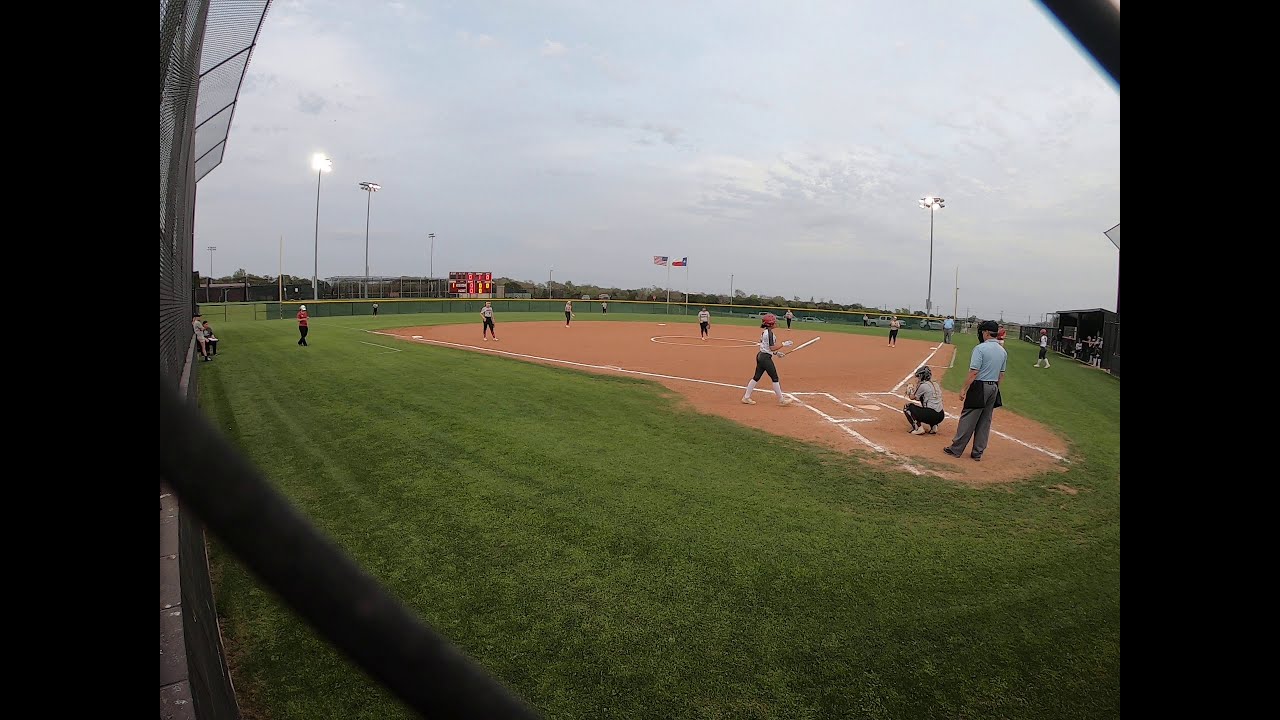The photograph captures a high-quality, horizontally aligned, rectangular image of a softball field taken from behind a black railing, possibly inside the bullpen. In the foreground, there is a neat expanse of green grass leading to the brown dirt of the infield, marked with white chalk lines defining the bases and home plate. Positioned at home plate is a catcher, donning black pants, a helmet, and a gray shirt. Behind her stands the umpire in gray pants and a short-sleeve light blue shirt, his face shielded by a black mask. A batter, dressed in a red helmet, white shirt, and black pants, is making her way to the batter's box. 

In the midground, distant outfield players can be seen wearing similar gray short-sleeve shirts. The scene is depicted under a hazy, clouded sky that remains light, suggesting an early evening setting as the stadium lights in the outfield have been turned on. In the background, two flags—likely the American and Texas flags—are visible, adding a sense of locale. Fencing on the far left side separates the field from the stands, where some trees and structures are discernible.